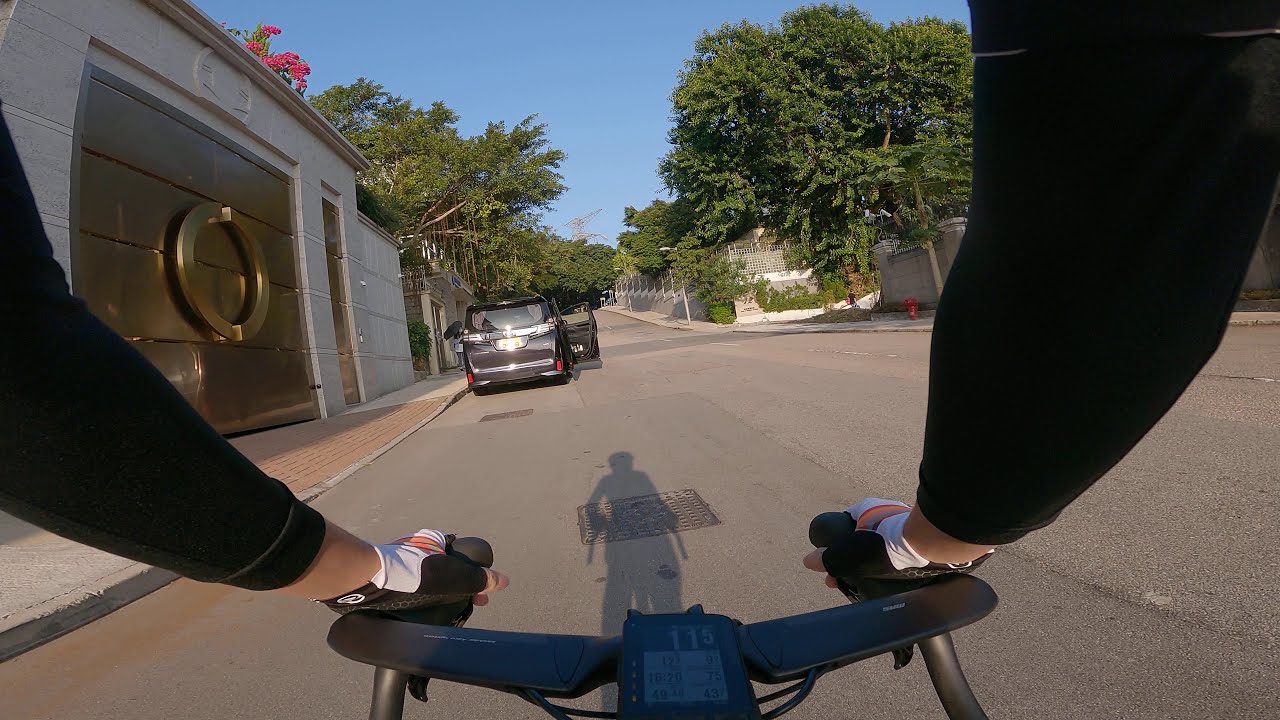This image captures the perspective of a bicyclist riding through a residential street. Taken from a chest-mounted camera, the photo reveals the rider's extended arms gripping black handlebars that curve inward, while they wear a snug black, long-sleeved shirt and white fingerless gloves. The digital speedometer on the bike indicates they are moving at 11 kilometers per hour. Directly ahead, a black minivan with its passenger door open is parked next to the sidewalk where a pedestrian stands under a black umbrella. To the left, a luxurious home features a striking golden gate with a large circular handle. The right side of the road is lined with barrier walls, probably marking another residential area, and tall trees dot the landscape. The sun is shining brightly behind the cyclist, casting long shadows in front of them on the clear day with a blue sky and no clouds.